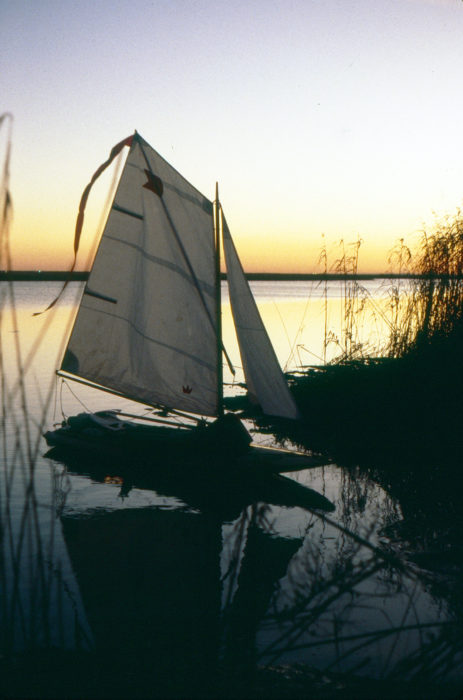The image depicts a small kayak with white sails, set in a natural, outdoor environment. Although the photo quality is somewhat blurry and low-resolution, the kayak is clearly distinguishable, positioned near the edge of a large body of water, possibly a lake. The backdrop features a striking sky with a gradient of colors: a pale violet-blue at the top, transitioning to a gold hue near the horizon. The kayak sports an intriguing detail—a white flag, potentially bearing a crown logo at the bottom right. Surrounding the kayak are silhouettes of dark banks and tall grasses, with plant life visible on both the left and right sides of the image. The scene, illuminated by bright lighting, lacks any visible inhabitants on the boat, presenting a serene, empty vessel in a tranquil, natural setting.